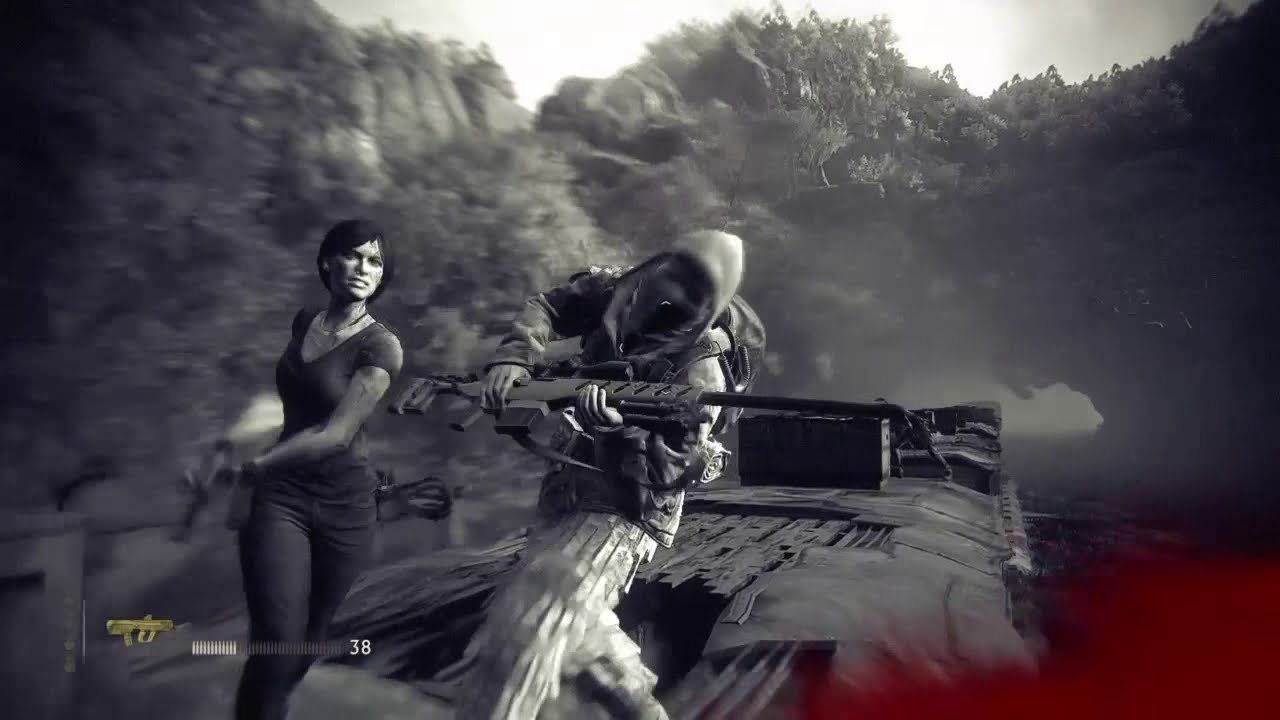This black-and-white screenshot from a video game captures an intense moment mid-fight on top of an old train winding through a rocky canyon. The scene shows a female protagonist, dressed in a short-sleeved V-neck shirt and jeans, forcefully striking a masked soldier with the stock of her gun. Her opponent, wearing a hoodie, backpack, and white camouflage pants detailed with ribbon-like materials resembling shrubbery, and holding a long rifle, appears to be reeling from the blow. The environment around them is detailed with rocky cliffs and sparse trees in the background. At the bottom of the image, there is a blood-like splatter effect, possibly signifying damage, along with a HUD element displaying 38 bullets remaining in the woman's machine gun. The action suggests this could be either a gameplay moment or a cutscene from a third-person shooter game.